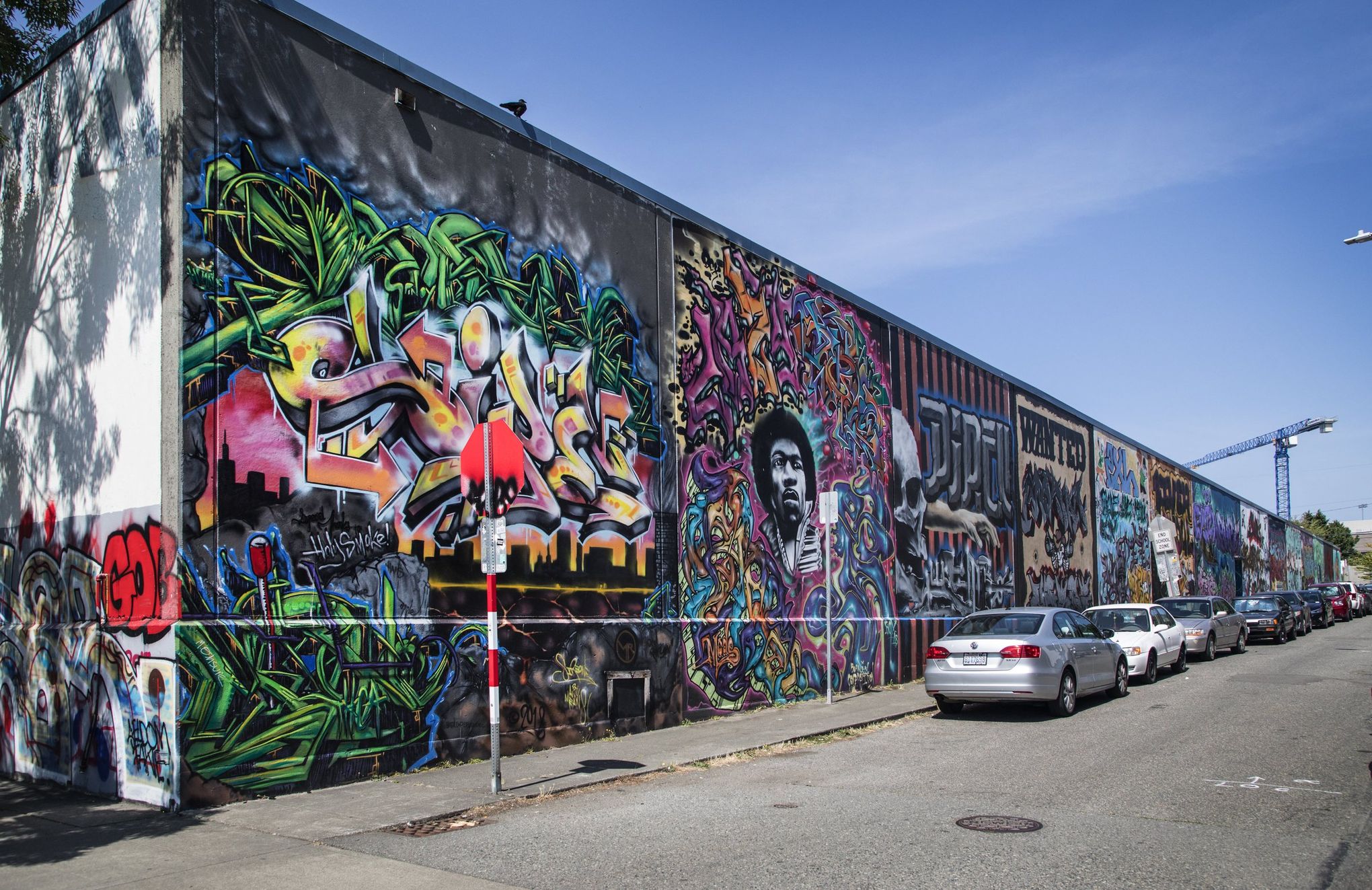In this vibrant street view, a warehouse-style building dominates the scene, adorned with colorful and intricate mural graffiti that spans its entire length. The graffiti panels feature diverse artwork, including a striking image resembling Jimi Hendrix, a skull, and a "wanted" poster, gradually becoming more indistinct as they recede into the distance. The foreground reveals a bustling urban street lined with parked cars running in both directions on the same side, adjacent to a sidewalk. A lone tree on the left and its substantial shadow are cast against the building, while a solitary bird perches atop the graffiti-coated structure. The bright blue sky is mostly clear, save for a single wispy cloud. Adding to the urban landscape, a blue crane looms in the distant background, and a stop sign, also defaced with graffiti, stands prominently in the forefront. Two manholes punctuate the road, contributing to the industrial atmosphere of the scene.